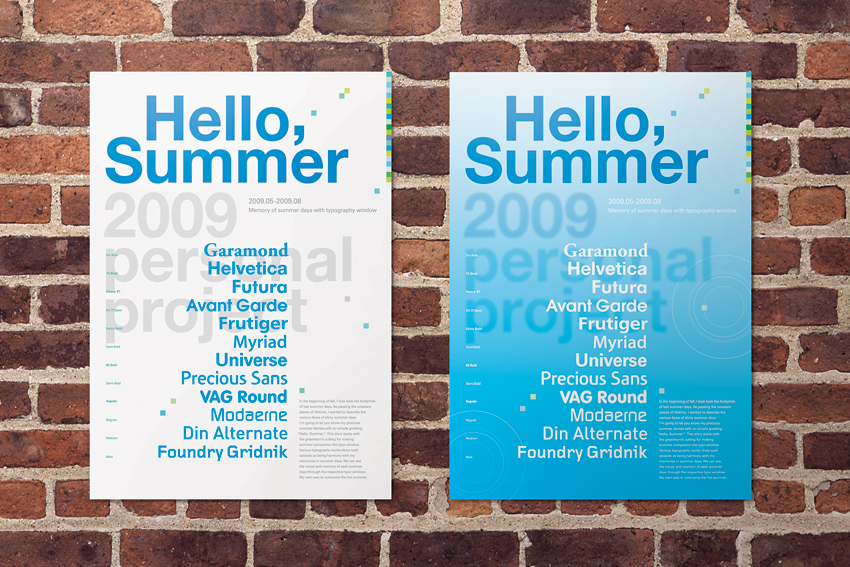This is a picture of two horizontally aligned posters mounted against a red brick wall. The poster on the left is white with blue letters, and the one on the right transitions from light blue to dark blue, featuring white text. Both posters prominently display the words "Hello Summer" in blue at the top, followed by "2009 Personal Project," which appears in gray on the left poster and in a faded blue on the right. In the center of each poster, a vertical list of font names is provided—blue text on the left and white on the right. The font names listed are Garamond, Helvetica, Futura, Avant-Garde, Frutiger, Myriad, Universe, Precious Sands, Vaground, Modern, Den Alternate, and Foundry Gridnik. Despite their different color schemes, the posters are identical in content, presenting an array of fonts in a visually engaging manner.